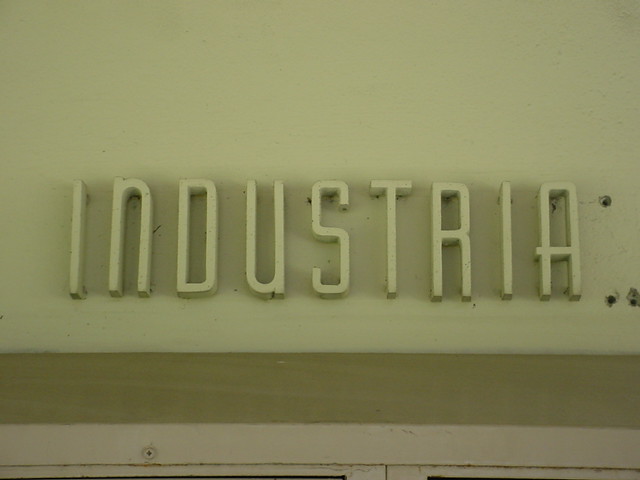The image depicts a white wall on a building structure, taken from a slightly elevated angle. The wall features large, three-dimensional, bold capital letters that appear to spell out "INDUSTRIA." The last letter "L" is missing, leaving behind three visible holes in the wall where it once was, indicating where screws or mounting points used to be. The creamy white letters blend subtly into the off-white background of the wall. Below the lettering, there are hints of a metallic window sill, suggesting that the letters are situated directly above a window or a series of windows. The overall scene includes no other visible objects or markings.